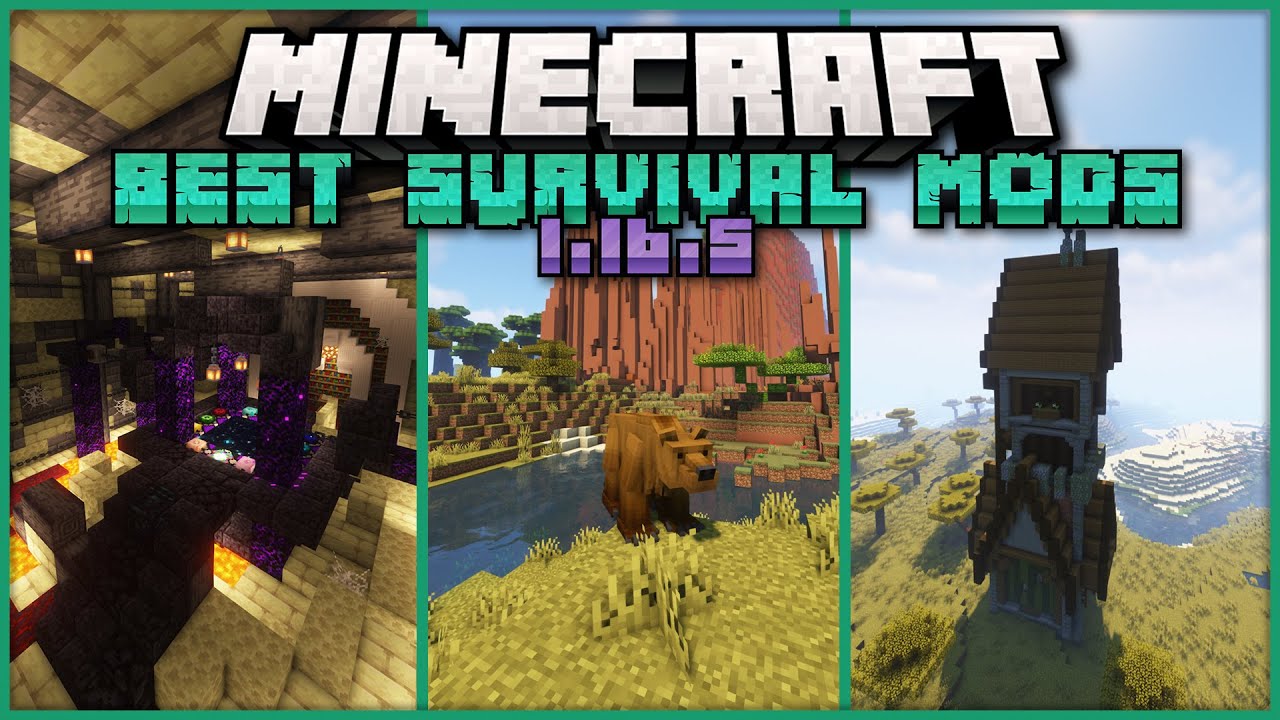This is a detailed poster for Minecraft titled "Minecraft Best Survival Mods." The title appears at the top in bold white letters, with "Best Survival Mods" highlighted in teal, and the version "1.16.5" displayed in purple. The poster is divided into three panels, each showcasing different Minecraft setups.

The left panel features an elaborate, dark room filled with various sophisticated Minecraft electronics and a well-lit dark table area, highlighting an intricate build. The middle panel presents a nature scene with a brown bear standing near a pond, surrounded by a mountainous landscape and lush trees, showcasing the wildlife additions. The right panel displays a tall, slender house resembling a treehouse, perched on a hill with a picturesque backdrop of mountains, green grass, blue sky, and scattered clouds. The overall theme suggests setups that enhance survival gameplay, potentially from a modding community.